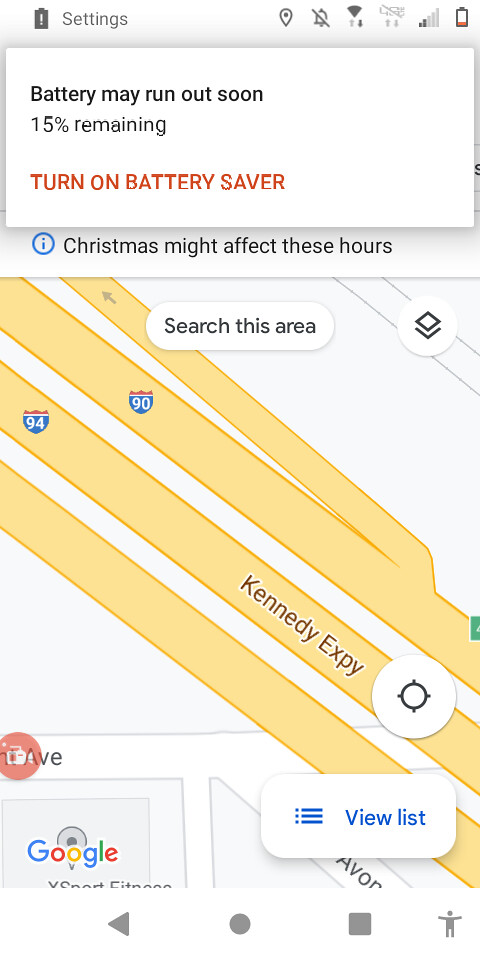A detailed screenshot captures various elements from an iPhone or similar smartphone. At the top of the screen, the heading reads "Settings". Several icons are displayed below, and one of them is a muted bell icon, indicating that the sound is turned off.

Just beneath the icons, a prominent notification warns, "Battery may run out soon, 15% remaining," with an option to "Turn on battery saver" highlighted in red. An additional note states, "Christmas may affect these hours," though the context is obscured by the battery alert.

The lower portion of the image transitions into a Google Maps section focusing on the Kennedy Expressway (EXPY). The expressway has four lanes on the upper left-hand side of the map, which converge into three lanes toward the lower right-hand side. Interstate 90 and Interstate 94 are marked with blue background signs above the lanes. Additionally, the label "Avenue" is partially visible along with the partial text "Google," indicating the map's source. On the right side, a "View list" option is shown in light blue. Additional minor icons appear at the bottom of this section, contributing to the interface's interactive options.

The screenshot clearly illustrates a blend of phone settings, battery notifications, and navigation details from Google Maps.